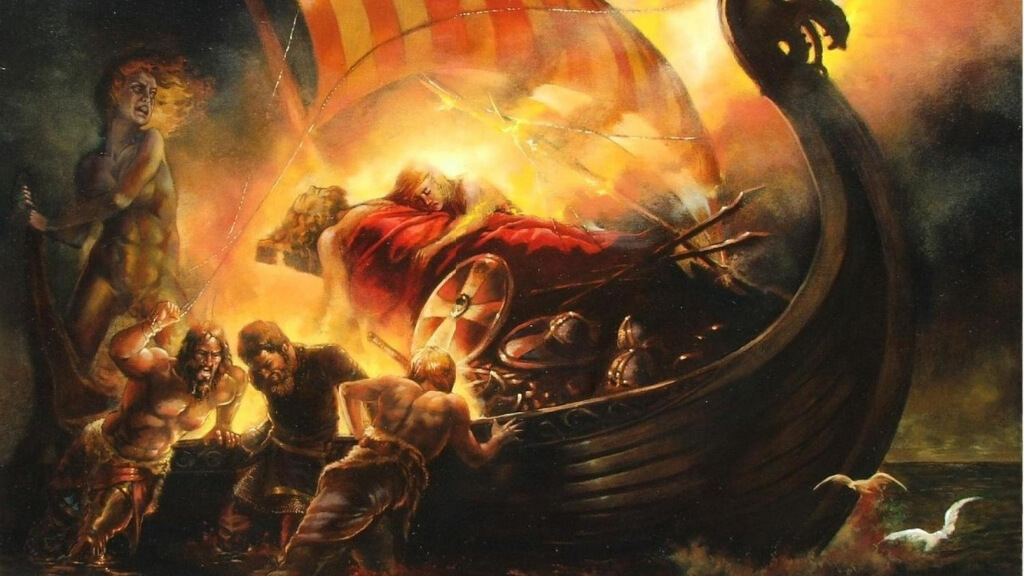The painting depicts a dramatic and tragic scene in a Renaissance style, filled with rich symbolism. At its center is a Viking longship, its dragon-headed prow rearing high and its wooden structure glowing fiercely from an intense blaze. Amid the flames, the boat is a chaotic sight of raw emotion. Men, shirtless with minimal attire, desperately push and wade through the surrounding waters, while their faces mirror the terror and anguish of the moment. A striking figure, possibly a woman—with long, wavy hair lit by the fire, and bare except for a hint of muscular definition—clings to the side of the vessel. Within the inferno-lit boat lies a man on a platform, his body solemnly draped in a red blanket. Another figure is tearfully draped over him, clutching his chest in grief. The scene is replete with Viking helmets and shields adorned with crosses, and a red and yellow striped sail stretches above, its colors contrasting sharply with the surrounding ocean on the right. This painting not only portrays a tragic incident but does so with profound emotional depth and intricate detail.